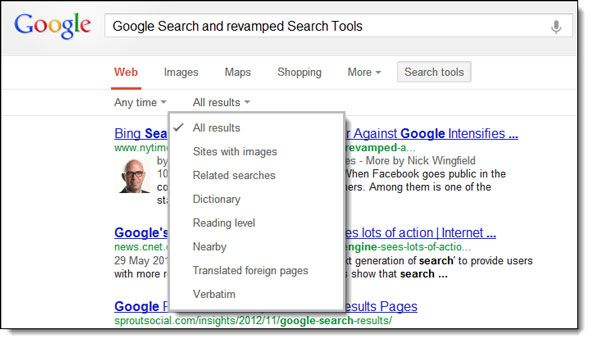The image depicts a computer screen displaying the Google search page. Dominating the top portion of the screen is Google's iconic logo in blue, red, yellow, and green letters. Directly below the logo is the search bar, which prominently features the text "Google search" accompanied by revamped search tools. Encasing the search bar is a gray banner.

Underneath the banner, there are six navigation choices: "Web" (highlighted with a red underline), "Images," "Maps," "Shopping," "More," and "Search tools." Below these options, an inset box is displayed. This box contains a menu titled "All results," which is checked. The menu lists several filtering options: "Sites with images," "Related searches," "Dictionary," "Reading level," "Nearby," "Translated foreign pages," and "Verbatim."

The inset box overlays part of the page's search results. Behind the box, some text is visible—appears to be the beginning of a search result titled partially with "Bing, S-E-A" in blue text, followed by "against Google intensifies." This partial title is accompanied by an image of a bald-headed man wearing glasses. Further down, hints of another title beginning with "Googles" can be seen, but the full context is obscured.

The background also includes various text snippets and some green and black writing. At the very bottom of the image, "Google" appears again in blue alongside "results pages." Further down is text indicating "sproutsocial.com insights 2012 Google search results."

Overall, the image is a snapshot of a busy Google search results page with several elements and options visible, presenting a typical view of a user's search experience.